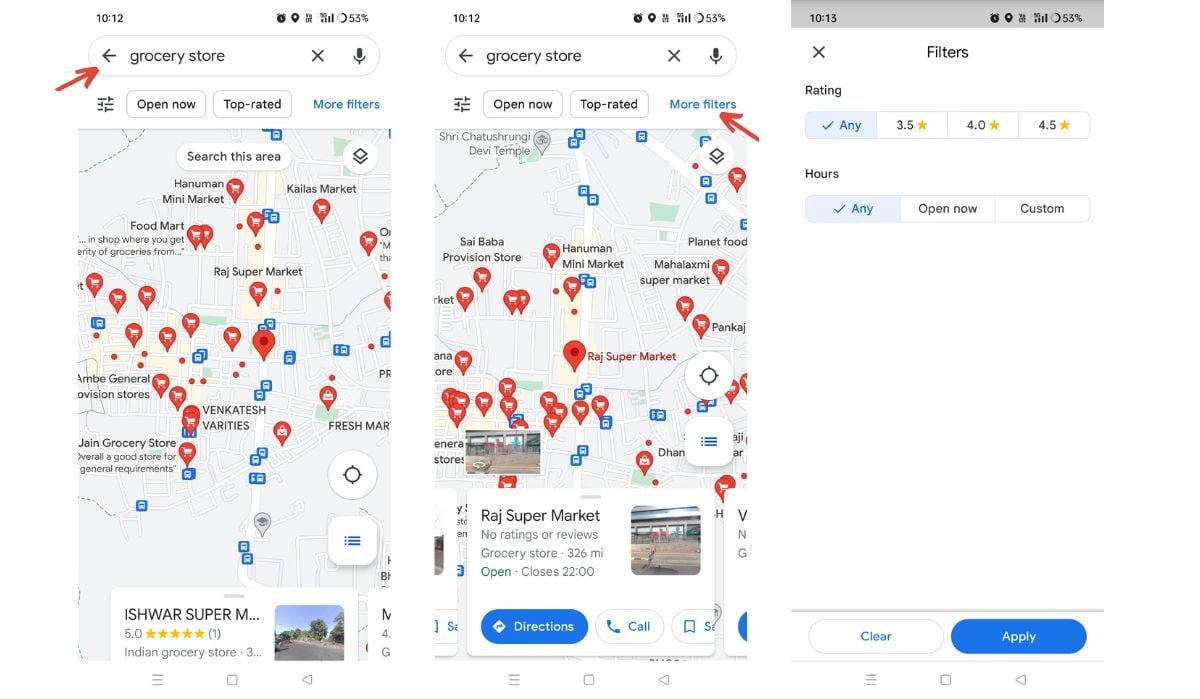This image comprises three distinct panels, each simulating a sequence of search results on a smartphone screen. 

**Panel 1:** The top of the screen displays the time "10:12" in black print, accompanied by standard phone status icons on the right—an alarm, location services, Wi-Fi signal, cellular signal, and a battery indicator showing 53% charge. Below this, a search bar contains the text "grocery store" with a red arrow pointing to it. To the left of the search term is a back arrow, and to the right, an 'X' and a microphone icon. Beneath the search bar, the options "Open Now," "Top Rated," and "More filters" are listed, followed by a map with various markers indicating grocery store locations. At the bottom, there is a highlighted result: "Ishwar Supermarket," rated 5.0 from one review, categorized as an Indian grocery store.

**Panel 2:** Similar to the first, but focusing on another grocery store search. The top of the screen remains unchanged with the time "10:12" and identical status icons. Below, the screen shows the search term "grocery store" with filters. A red arrow is pointing towards "More filters." At the bottom, a result for "Raj Supermarket" (spelled Rej) appears, with options to view that it is open, get directions, or call.

**Panel 3:** The top panel's time updates to "10:13," with nearly identical status icons. The main focus of this panel is filter options. A grey banner at the top says "X Filters" with a court symbol in the center. The filter options include rating categories (3.5, 4.0, or 4.5 stars). The "Any" option is selected. Additionally, there are options for hours ("Any," "Open Now," "Custom"), with "Any" being selected for hours as well.